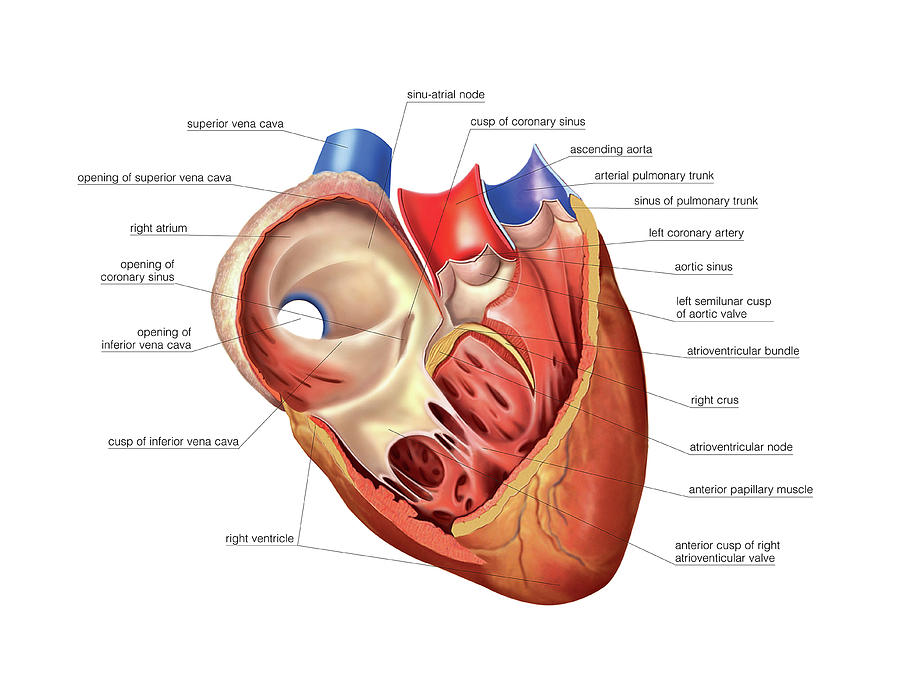The image is a highly detailed anatomical chart of the human heart set against a white background, designed for educational purposes. It features a color-coded illustration of the heart, including a cross-section that reveals the internal structures and different types of tissue. The chart meticulously labels various parts of the heart with thin, dark lines connecting to text annotations. These labels include the sinuatrial node, superior vena cava, opening of superior vena cava, right atrium, opening of coronary sinus, inferior vena cava, right ventricle, anterior cusp of right atrioventricular valve, anterior papillary muscle, atrioventricular node, right crus, atrioventricular bundle, left semilunar cusp of the aortic valve, aortic sinus, left coronary artery, sinus of pulmonary trunk, arterial pulmonary trunk, and ascending aorta. The diagram uses color coding to highlight different anatomical features, with veins depicted in blue, arteries in red, and other areas in varying shades of brown, cream, and yellow.